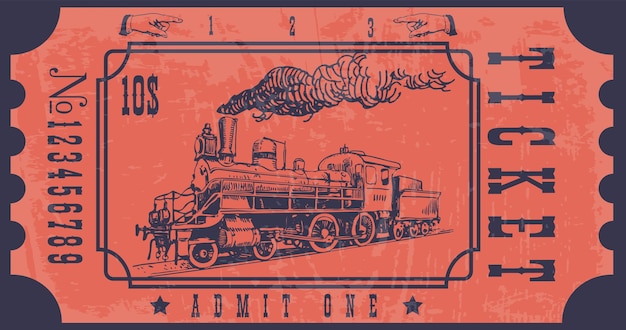This image features a digitally created depiction of a vintage train ticket against a black background. The ticket itself is orange and enclosed in a rectangular black frame. Prominently, in the center, there is a black and white illustration of an old-fashioned steam train billowing smoke as it moves leftward from the right side of the ticket. Above this illustration, aligned with the upper left corner, is a "$10" mark. Just above this section are the numerals "1 2 3" flanked by a pair of hands—one to the left of the "1" and one to the right of the "3"—both pointing inward. On the left vertical edge of the ticket, the numbers "1 2 3 4 5 6 7 8 9" are written in black. Beneath the train, at the bottom center, the text "ADMIT ONE" is prominently displayed between two black stars. Lastly, the word "TICKET" is positioned vertically on the far right of the ticket in large, bold black letters.